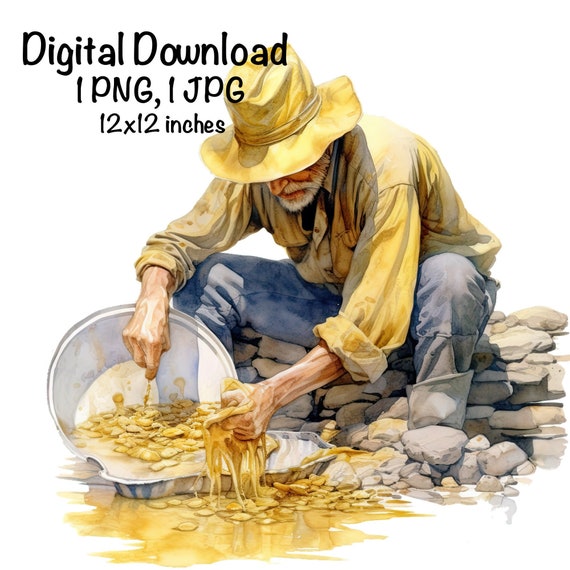This is a detailed painting, evoking the style of either watercolor or acrylic, featuring an old-time prospector panning for gold in a river. The focus is on an elderly white man with a scruffy white beard and mustache, his eyes obscured as he looks down towards his gold pan. He wears a worn, tan wide-brimmed hat and a yellow long-sleeved, button-down shirt with the sleeves partially rolled up to reveal his forearms. His attire also includes blue denim jeans and gray boots, though the bottom of the boots is not visible. The man sits on a stone wall with a metal pan in one hand and a washcloth in the other, with water dripping from it. In front of him, a tin dish sits, possibly containing rocks and other materials sifted from the river. A watermark is visible in the top left corner, reading "digital download, png, jpg, 12x12 inches". The overall scene captures the essence of historical gold mining in a serene, painterly fashion.